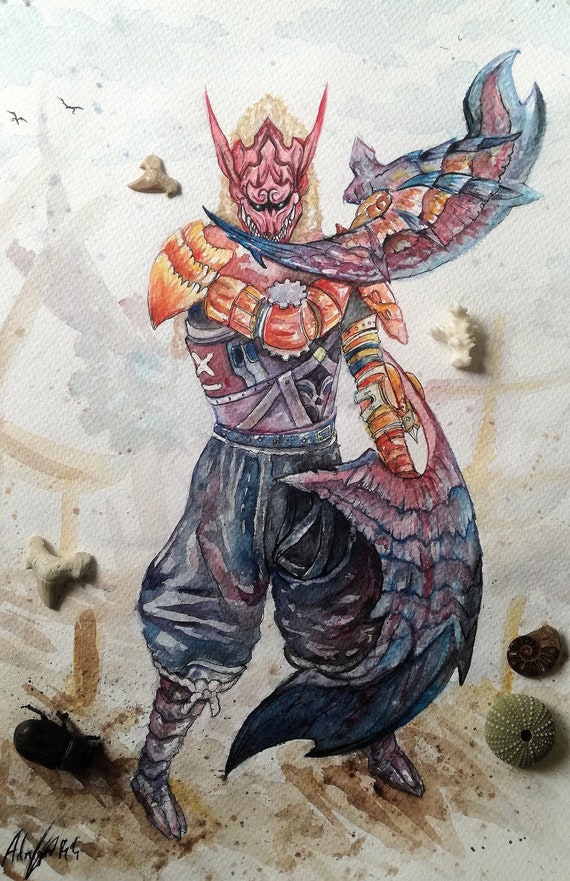This mixed-media fantasy painting, crafted on a canvas, features a striking demon warrior as its central subject. The background is a gradient of bluish watercolors at the top, transitioning to brown brushstrokes at the bottom. Surrounding the figure are glued objects, including a small round cactus-like plant, a large black water bug on the left, small bone-like plaster pieces on both sides, a shell, and two shark teeth, giving the artwork a three-dimensional quality.

The creature, set against a textured backdrop with shades of purples, browns, tans, and blues, wears long black baggy pants that balloon at the knees and brown knee-high boots that tie with a white bow. Its upper body is adorned with a metal chest guard featuring a white 'X' on the side and a red and purple sash. The creature's arms are shielded with orange armor extending from the shoulders to the wrists, resembling feathers or wing-like structures with spikes. The hands are similarly adorned with long feathers.

The warrior's face is concealed by a red dragon-like mask with long, pointy ears and jagged fangs, and blonde hair flows beneath the mask. The overall scene is punctuated by an illegible signature at the bottom, hinting at the artist's identity. This piece masterfully blends watercolor with tactile elements, creating a vivid and immersive portrayal of a fantastical demon warrior.